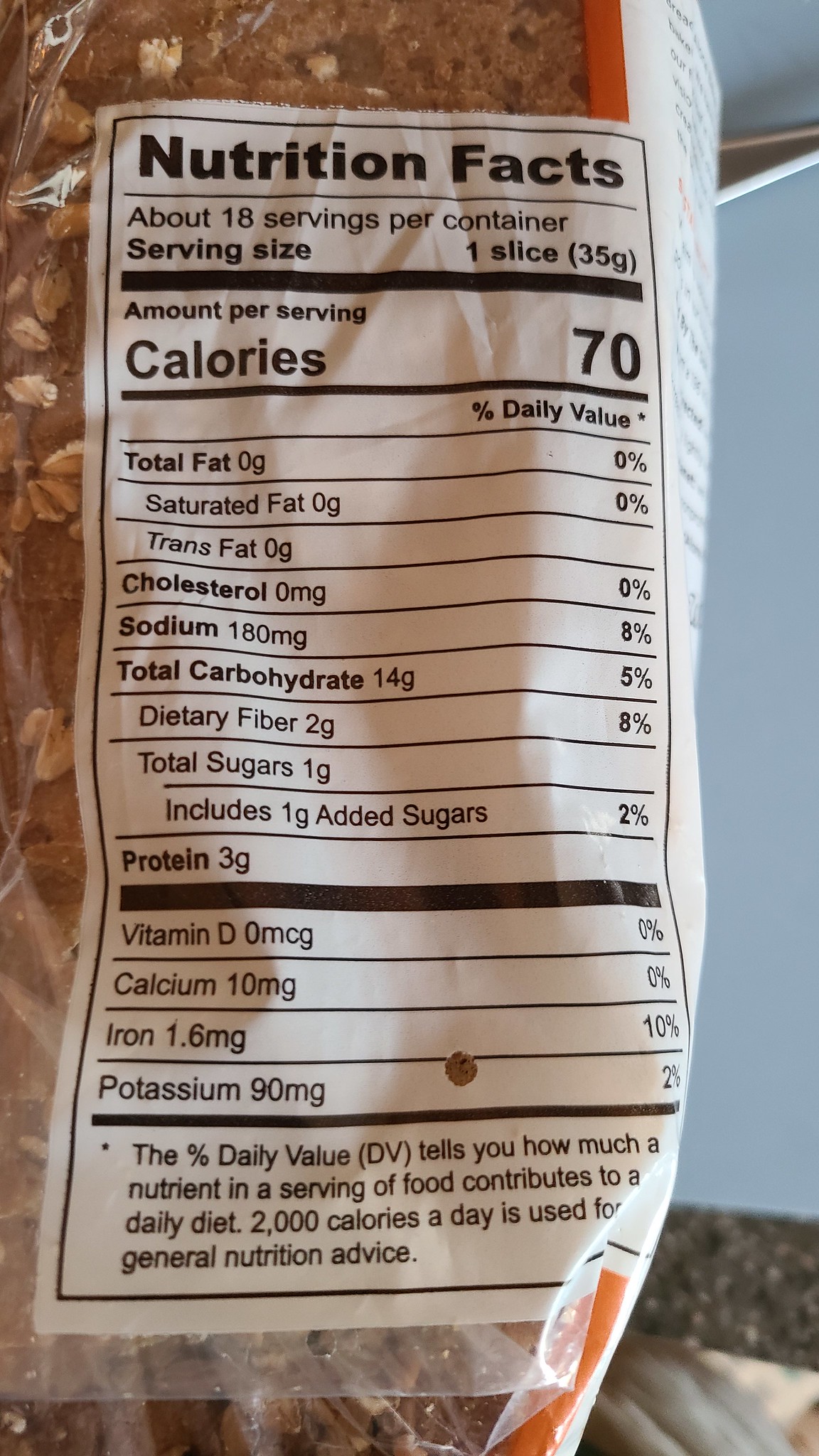This image shows the nutrition facts label of what appears to be a loaf of whole grain bread. The label indicates that the loaf contains approximately 18 servings, with each serving size being one slice, or 35 grams. Nutritional information per serving is detailed as follows: 

- **Calories:** 70
- **Total Fat:** 0 grams (0% DV)
  - **Saturated Fat:** 0 grams (0% DV)
  - **Trans Fat:** 0 grams
- **Cholesterol:** 0 milligrams (0% DV)
- **Sodium:** 180 milligrams (8% DV)
- **Total Carbohydrate:** 14 grams (5% DV)
  - **Dietary Fiber:** 2 grams (8% DV)
  - **Total Sugars:** 1 gram 
    - **Includes Added Sugars:** 1 gram (2% DV)
- **Protein:** 3 grams
- **Vitamin D:** 0 micrograms (0% DV)
- **Calcium:** 10 milligrams (0% DV)
- **Iron:** 1.6 milligrams (10% DV)
- **Potassium:** 90 milligrams (2% DV)

The label also notes that the percentage Daily Value (DV) indicates how much a nutrient in a serving of food contributes to a daily diet, with a general guideline of 2,000 calories per day for overall nutrition advice.